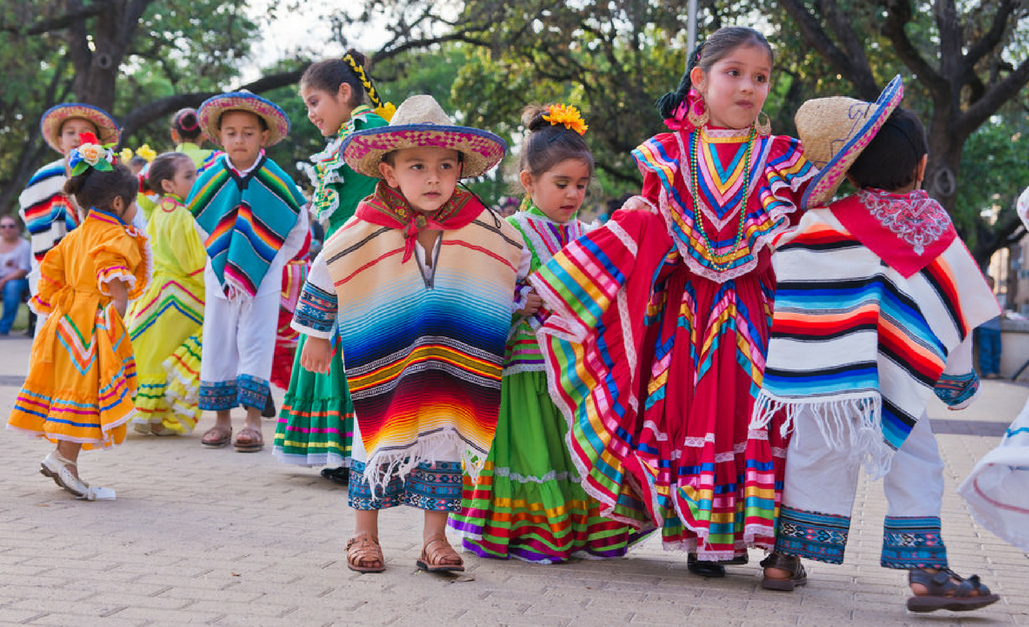The image captures a delightful outdoor scene of 11 or more little children celebrating Cinco de Mayo. They are dressed in vibrant traditional Mexican attire: the boys in colorful striped ponchos and sombreros, and the girls in equally vivid dresses complemented with big flowers in their hair. The children are paired up, holding hands as they walk along a light gray brick sidewalk, with some playing or dancing. The setting appears to be a park or square, with a line of trees heavy with foliage in the background, adding to the festive atmosphere. The sky is visible above, casting a white glow over the scene, enhancing the overall cheerful and lively ambiance.